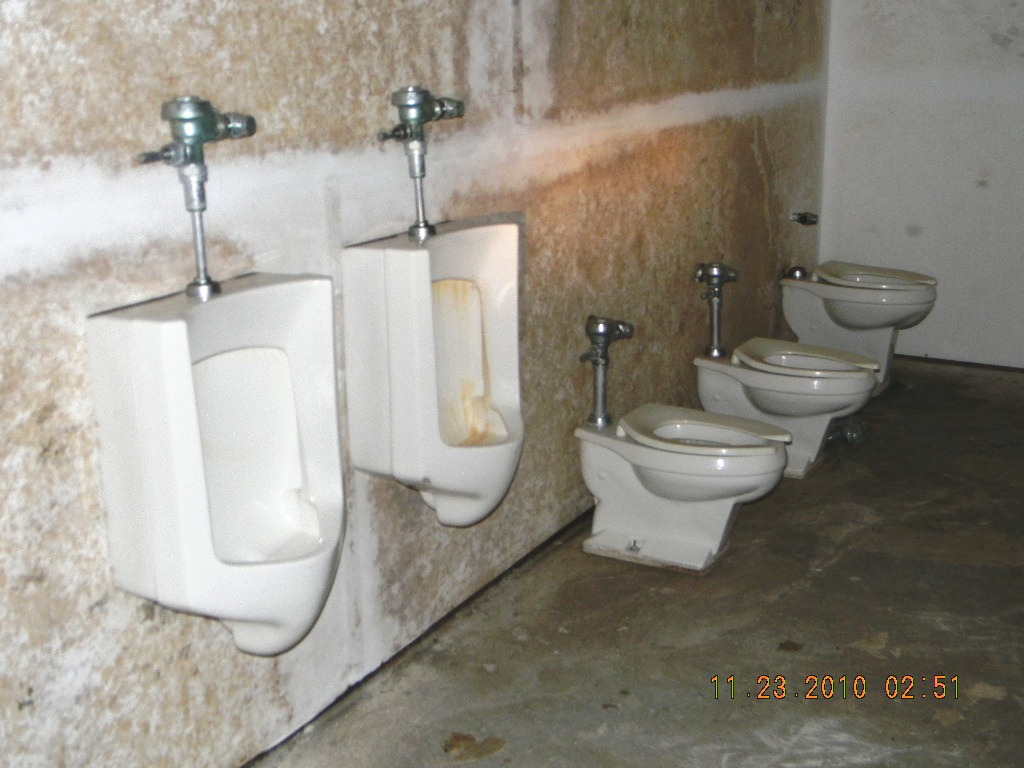The photograph captures a neglected and grimy public restroom, likely abandoned or in disrepair, featuring two white porcelain urinals on a concrete wall with no dividers between them. The left urinal appears relatively clean, while the right one is stained and dirty with a streaky yellow liquid. To the right of the urinals, three decrepit toilets are lined up against the wall, all with closed lids. The toilets and urinals are connected to a white and brown stained wall that looks unfinished. The entire room is characterized by its concrete floor, which is dirty and water-stained with shades of gray and brown, particularly darkening towards the back right. The wall has a rough concrete or drywall appearance with some white trim and visible brown spots. A date, "11.23.2010, 02:51," is marked in orange on the bottom right corner of the image, suggesting the time and date when the photo was taken. The room's overall unkempt and abandoned appearance is accentuated by its dingy, streak-ridden surfaces and peeling textures.